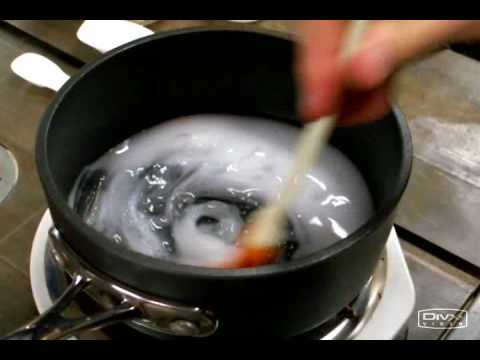This indoor image captures a high-angle view of a cooking scene, focusing on a black saucepan resting on a white burner with a silver rim. The pot holds a white, shiny substance being stirred by a hand emerging from the top right of the image, clutching a white handle with a red-orange tint. The hand and utensil appear blurry, making the utensil type indistinguishable. The black saucepan's position is central in the image, highlighting the transparent spots in the white paste and the visible black bottom of the pot. A barely readable brand name, possibly "DIVX" or "DIVA," is located at the lower right of the burner. The image features black borders at the top and bottom, seamlessly extending to the photo’s edges on the sides, emphasizing the intimate cooking activity within a kitchen environment.